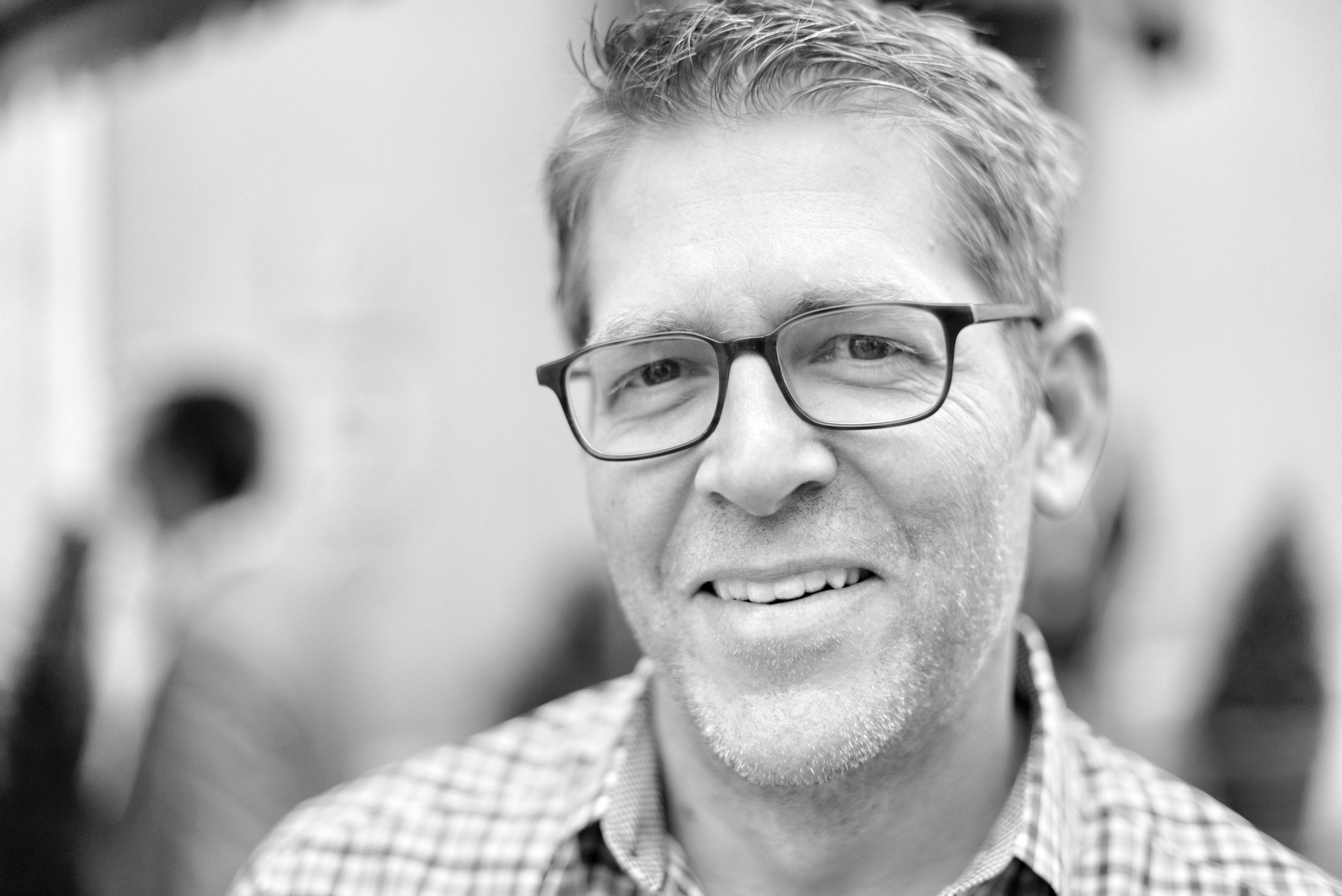In this black and white photograph, the central focus is a man looking directly at the camera with a sincere smile, showcasing his top teeth. He is wearing semi-round, black-rimmed glasses and a checkered shirt, where the pattern alternates between white and black. His hair is short, wavy, and combed towards the left side, with a bit of scruff indicating he hasn't shaved recently. The background is highly blurred, predominantly white with occasional dark areas, suggesting a wall or window behind the man, along with an indistinct figure to the left, possibly another person with dark hair. The image does not contain any text and appears to be set in a public place, though the exact setting remains indeterminate due to the blurriness of the background.